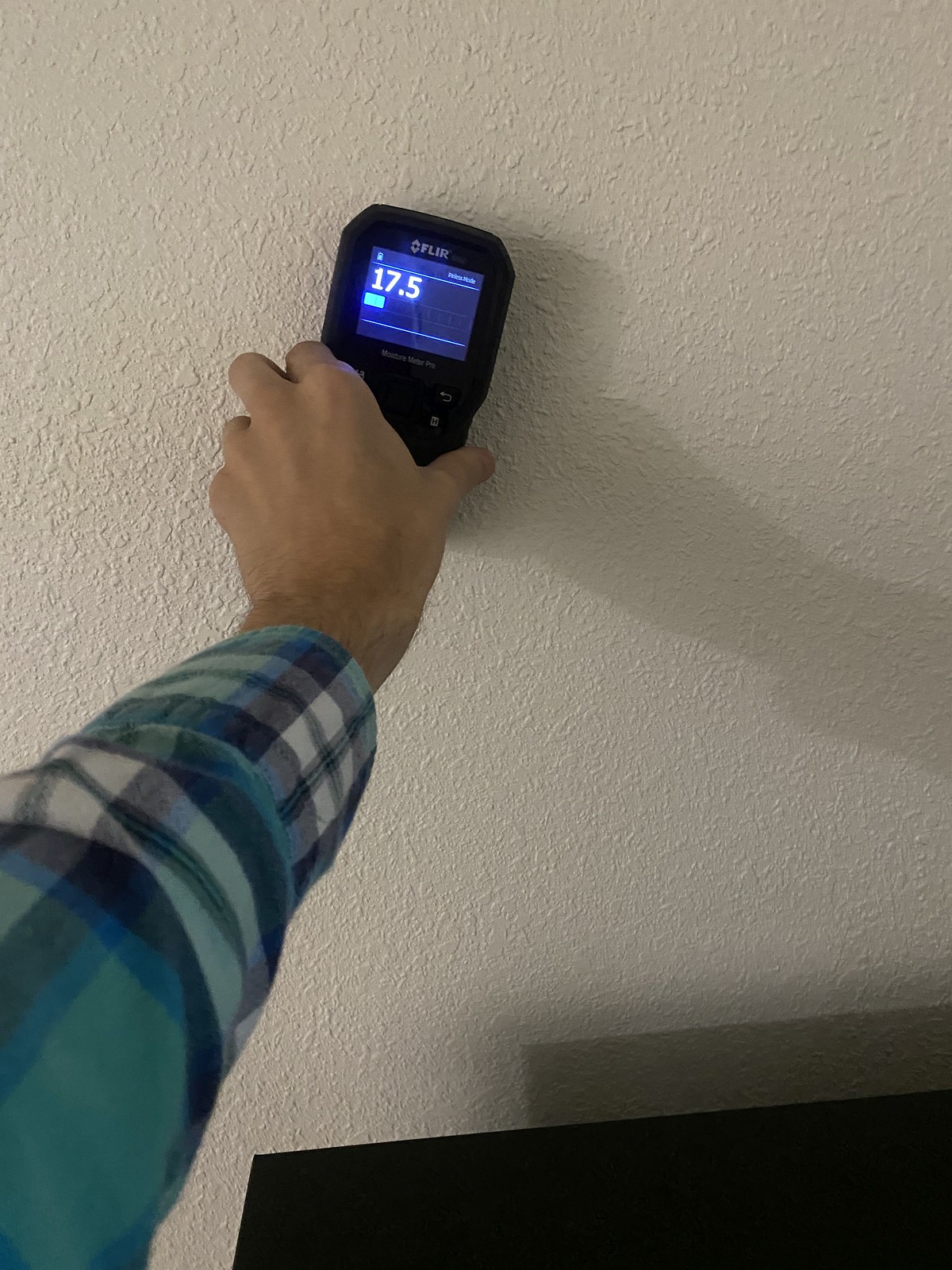In this detailed image, an arm clad in a long-sleeved, checkered shirt featuring a palette of light blue, dark blue, white, and possibly black, is prominently visible. The hand, emerging from the shirt, holds a black device noticeably marked with the brand name "FLIR" on its upper section. This device, which appears to be a specialized instrument used for readings, is held slightly tilted against a textured white wall. The screen of the device displays a numerical reading of "17.5", accompanied by a small blue bar located just below this number. In the lower right corner of the device's screen, a black shelf or table is faintly visible, with its reflection subtly mirrored on the wall, as is the person's hand gripping the device.